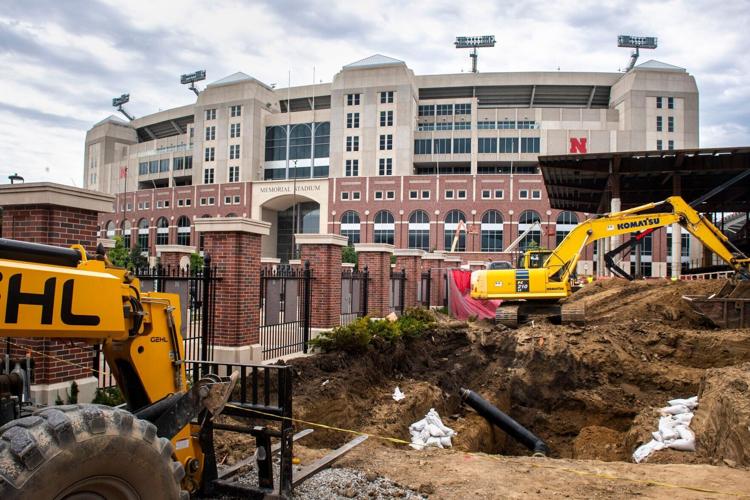The image depicts an active construction site where significant excavation work is being performed. Two bulldozers, one orange and one yellow with large black tires, have created a substantial pit in the dirt field. The pit is partially filled with green shrubs and small trees that remain amidst the soil. The entire site is enclosed by a combination of tall black metal fencing and robust brick walls, which form a perimeter around the area. The fencing and brickwork alternate in sections, providing sturdy security and a defined boundary for the construction zone.